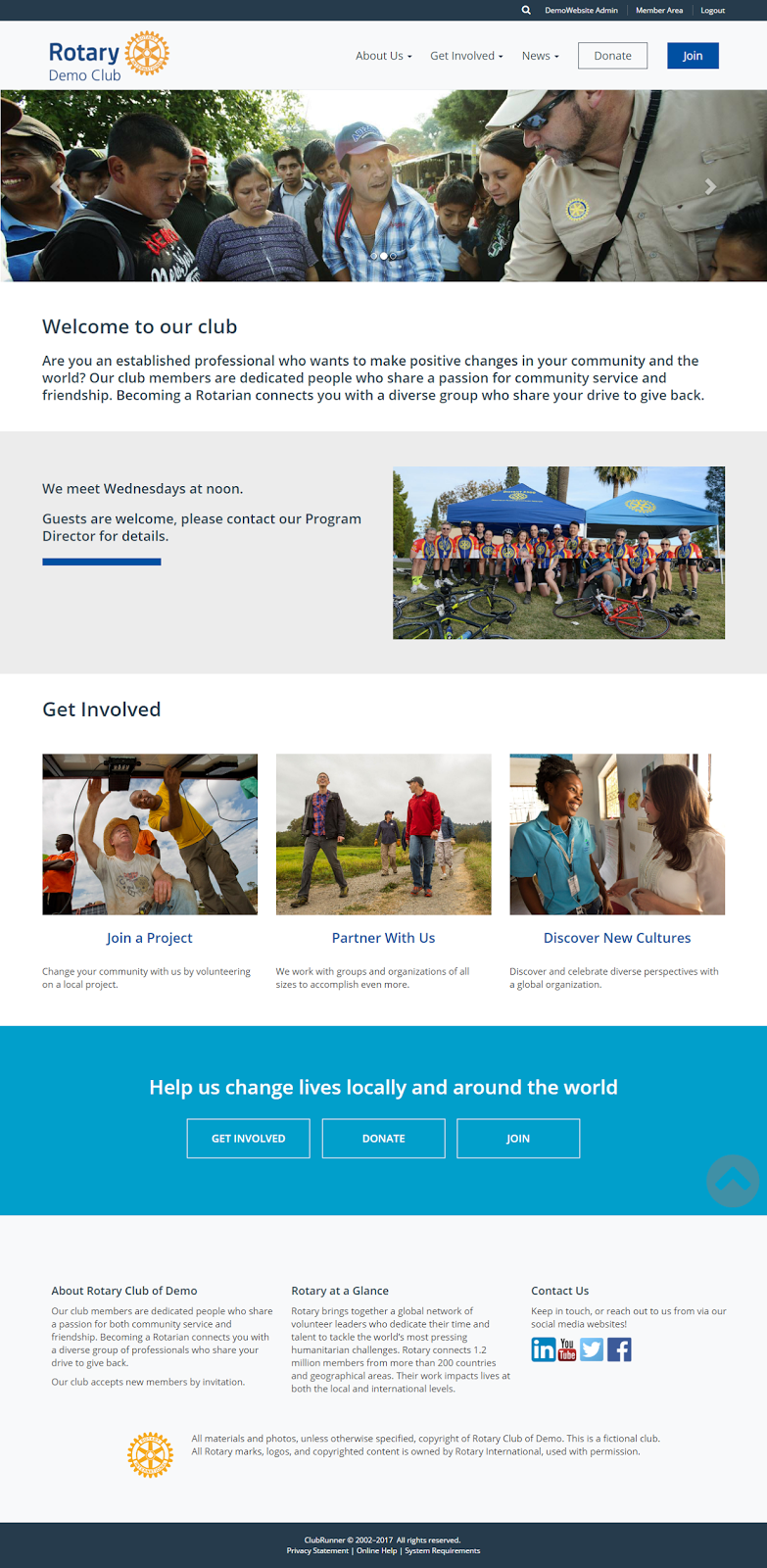The image showcases the homepage of the Rotary Demo Club on a cell phone screen. Prominently featured at the top is the club's name alongside an orange gear icon. Upon zooming in, several clickable areas become visible, labeled as "About Us," "Get Involved," "News," "Donate," and "Join," with "Donate" highlighted in white and "Join" in blue, each housed in their own marked rectangles.

Additional navigation options include "Members Area," "Demos Website Admin," and "Logout." A welcoming message invites viewers with the text: "Welcome to our club," accompanied by an image of a group of cheerful people, some looking down and smiling as sunlight illuminates the scene in the background.

The club promotes engagement with a message: "Are you an established professional who wants to make a positive change in your community and the world? Our club members are dedicated people who share a passion for community service and friendship. Becoming a Rotarian connects you with a diverse group who share your drive to give back."

Furthermore, the page indicates the club's meeting schedule: "We meet Wednesdays at noon. Guests are welcome. Please contact our program director for details." The newsletter content continues further down the page.